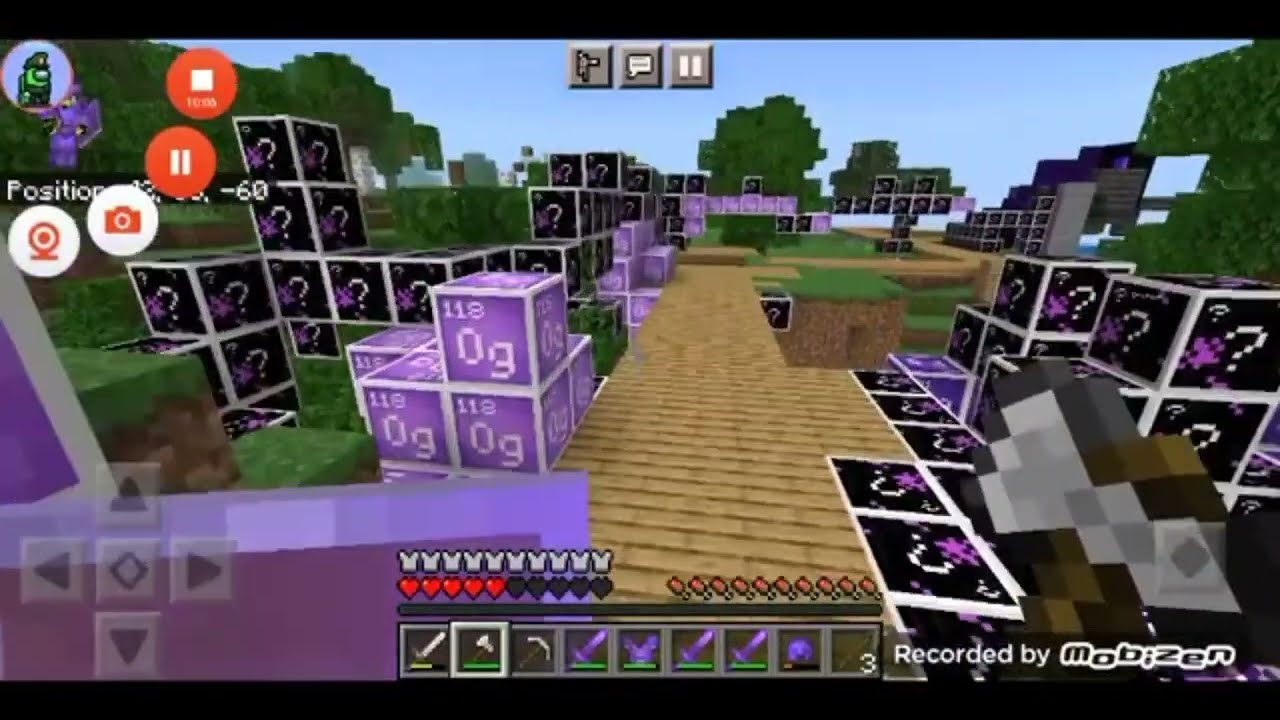In this detailed, descriptive caption, we'll consolidate the shared and unique details provided by each person to create a comprehensive image description:

---

This is a screenshot from a video game, widely resembling Minecraft, displaying a first-person perspective where the player appears to be navigating through a maze-like setting. The scene features a beige or wooden brick path running down the center, with the player holding an indistinguishable brown and white object in the lower right corner of the screen. On both left and right sides of the path are stacks of various cubes forming obstacles.

On the left side, there are lavender or purple cubes arranged two or three blocks high, resembling periodic table elements, specifically marked with '118' and 'OG'. Surrounding these and receding into the distance are black cubes adorned with pixelated white question marks. These black cubes also appear on the right side of the path alongside similar scattered stacks.

In the background, the landscape includes grassy terrain, trees, and a clear blue sky. At the bottom of the screen are several gameplay interface symbols, including red and black heart emojis, meat kebab emojis, and directional controls represented by grey triangles.

The bottom right corner of the image is overlaid with the text "Recorded by Mobizen," characterized by white letters with an uneven alignment. 

The player appears well-equipped, possibly preparing to solve puzzles or face potential enemies in this seemingly deserted maze-like world.

---